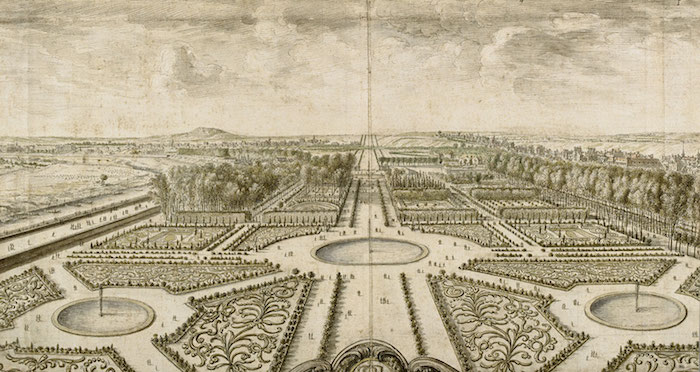A meticulous antique drawing rendered in brown ink on parchment paper, presented in a landscape orientation. The artwork showcases an expansive outdoor garden extending all the way to the horizon. The garden features elaborate and intricate designs, including an array of labyrinth-like pathways. Three prominent circular fountains are positioned distinctly: one in the center, and the other two in the left and right foregrounds. Scattered across the pathways are minuscule, finely-detailed depictions of people, further enhancing the complexity and depth of the scene. The level of detail in this drawing highlights the artist's masterful precision and dedication.